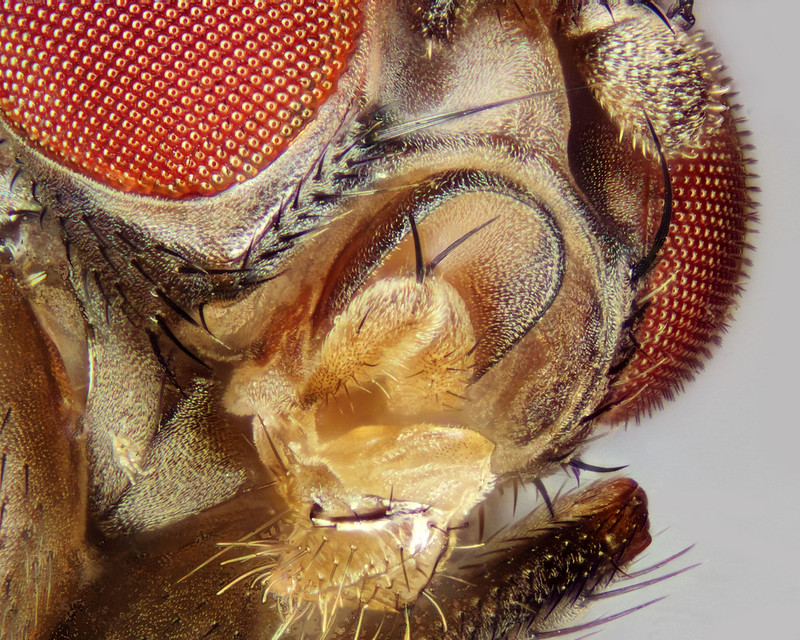This image is an extreme close-up, magnified photograph of a fly's face, showcasing intricate details that are difficult to discern at first glance. Dominating the upper left corner is the fly's reddish, multifaceted eye, which appears almost pixelated due to the detailed texture. The fly’s face, illuminated in shades of light brown, tan, and gold, features an array of hair-like protrusions extending from its mouth and jaw area, giving it a somewhat fuzzy appearance. Visible beneath the insect and viewed from an upward angle, the photograph highlights additional components, including parts of the thorax and another eye in the background. Central to the image is a yellowish mechanism, likely part of the fly's mouthparts, adding to the intricate complexity of the insect’s visage.